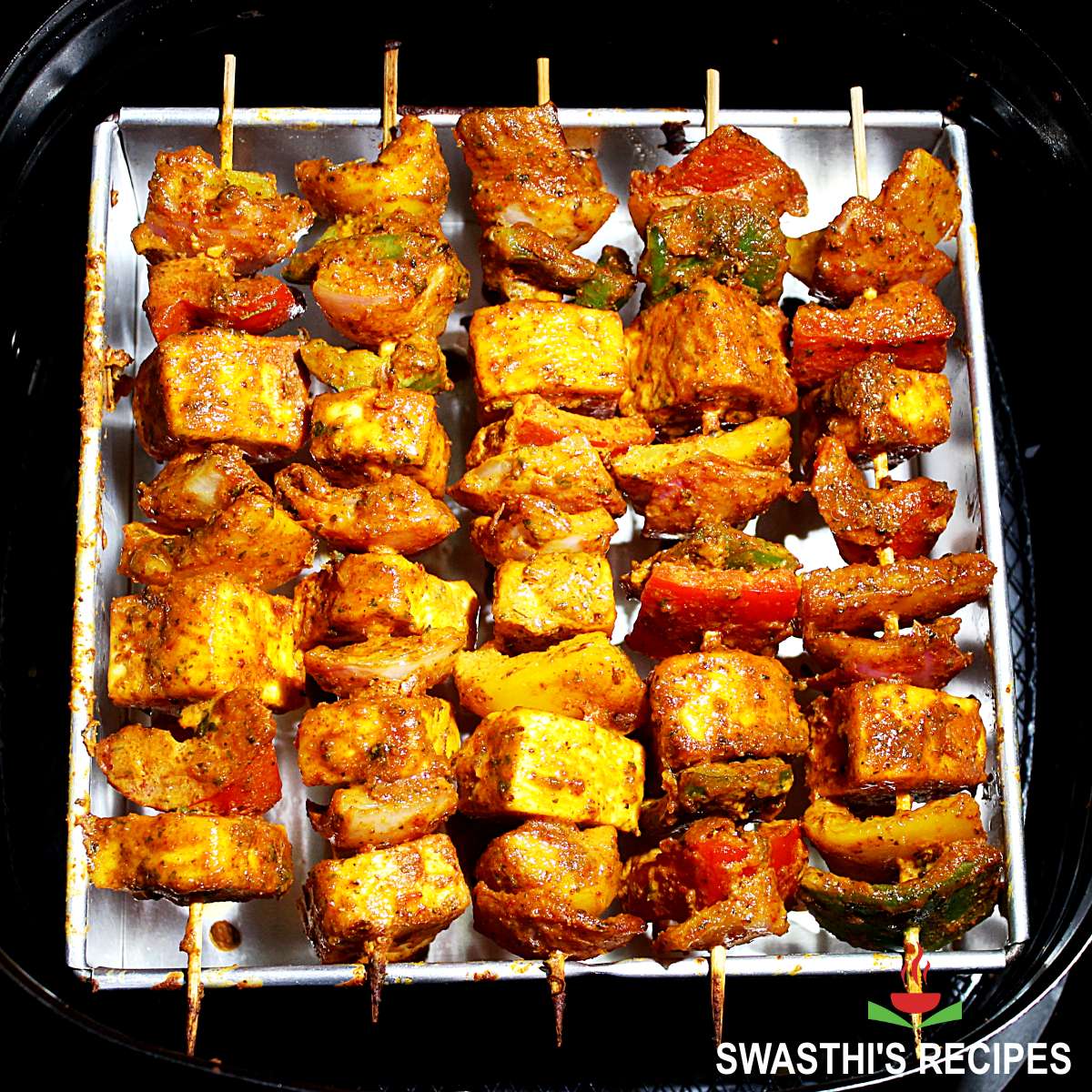The close-up image showcases five shish kebabs, each featuring large cubes of meat, potentially chicken or pork, accompanied by roasted red and green bell peppers. The kebabs are skewered on thin bamboo sticks and are arranged side by side, balancing horizontally over a smaller rectangular stainless steel tray. This smaller tray is nested within a larger round black tray. The meat appears yellow and orange, likely influenced by the lighting or sauce applied. A reddish-orange sauce coats the skewers, enhancing their vibrant appearance. At the bottom right corner of the image, the caption "Swasti's Recipes" is displayed in white font, with a decorative green and red design above it.